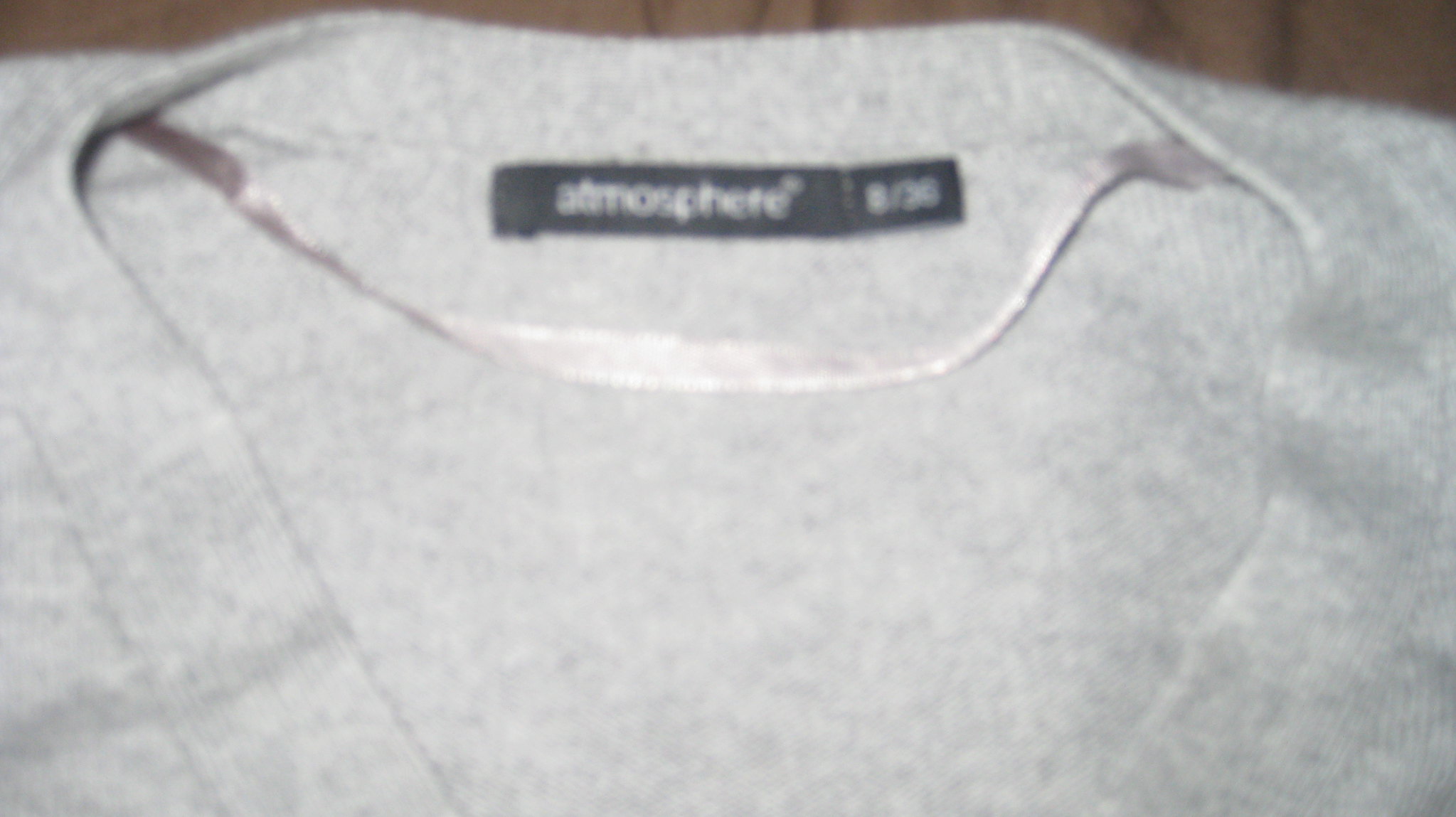The image depicts a close-up view of the neckline area of a gray shirt. The visible stitching around the neckline is neat and well-defined. There is a hole in the fabric for the head, as is typical for shirts. A dark-colored tag is positioned near the top of the collar line. Although the text on the tag is blurry, it appears to read "Atmosphere." Next to this tag is a smaller, dark tag with white characters that seemingly read "8/30," though the blurriness makes this hard to confirm. The shirt is resting on a wooden surface, characterized by a brown color with darker wood grain lines.